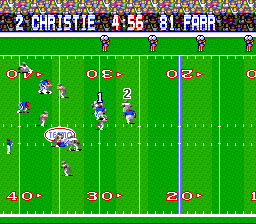This image is a screenshot from the classic Tecmo Super Bowl arcade game, likely from around 1990. The scene displays a football game between two teams, with one team in blue uniforms, and the other in what appears to be gray or silver and white uniforms. The view is slightly wider than it is tall, revealing a green football field marked with yard lines; the 40, 30, and 20-yard lines are visible, and the play is centered around the 30-yard line, where a field goal is being attempted. At the very top of the screen, the scoreboard information reads "2 Christie" and "81 Far," with a timer showing 4:56 left in the game. Above the field, a crowd of spectators is digitally generated, adding to the nostalgic atmosphere of this iconic sports video game. The Tecmo logo is also prominently displayed in the middle of the screen, reinforcing its classic arcade origin.